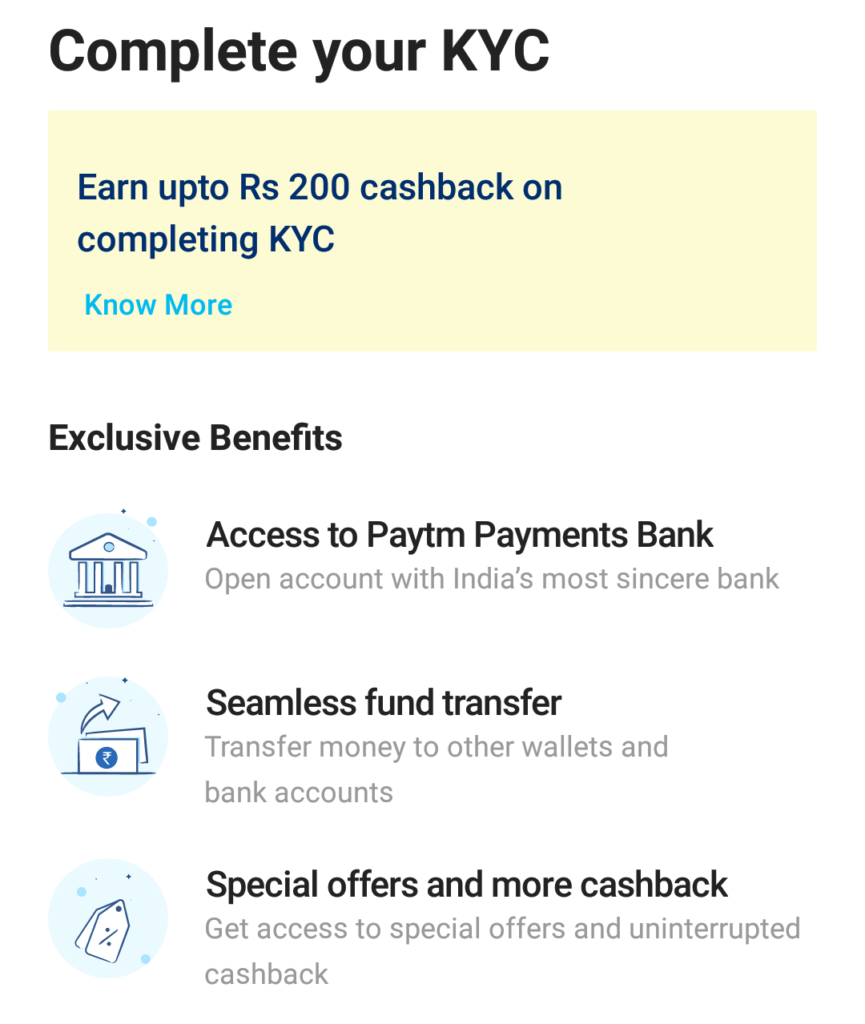Screenshot of a banking app interface displaying a prompt to complete KYC (Know Your Customer) verification. At the top of the screen, bold text reads, "Complete your KYC and earn up to Rs. 200 cash back on completing KYC." Below this, there is a mention of "Exclusive Benefits" accompanied by three icons. 

The first icon is of a bank, labeled "Access to Payments Bank." The second icon, resembling letters, is labeled "Seamless Fund Transfer." The third icon, featuring a tag, is labeled "Special Offers and More Cashback." The layout suggests a user-friendly design with incentives prominently highlighted to encourage KYC completion.